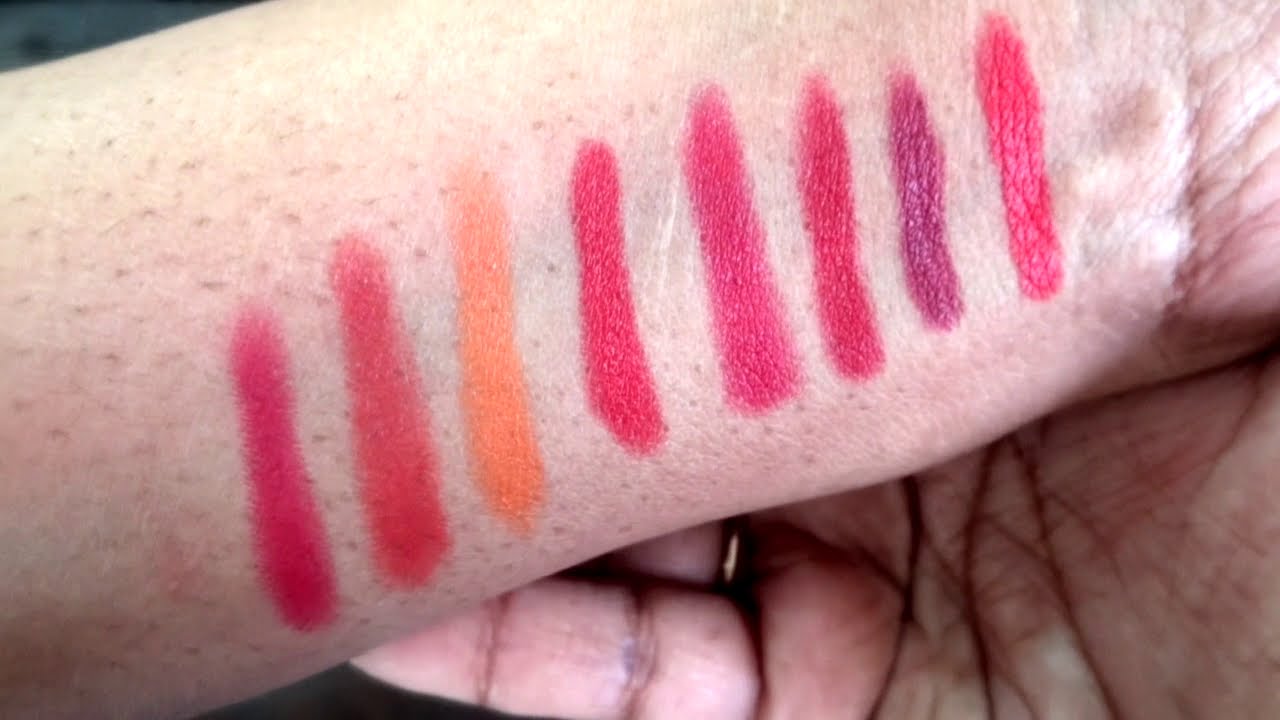This photograph in a landscape layout captures a close-up of a Caucasian person's arm, oriented diagonally across the frame. The arm showcases eight distinct color strips that likely represent swatches of lipstick. Moving from the bottom to the upper right, the colors transition from pink to orange, lighter orange, red, pink again, maroon, darker amber, and a light red. The arm, belonging to a person with white skin, is detailed with small black speckles, likely freckles or moles, and light hair. The presence of the right hand's palm in the bottom right corner, holding up the arm, adds an additional layer of interest. Only the pinky, partial ring finger adorned with a gold ring, and a hint of the middle finger are visible, showcasing the numerous wrinkles and lines of the palm. The background features a black triangular corner in the upper left, contrasting sharply with the arm and highlighting the texture and colors of the painted stripes in this meticulously detailed and intimate portrait.